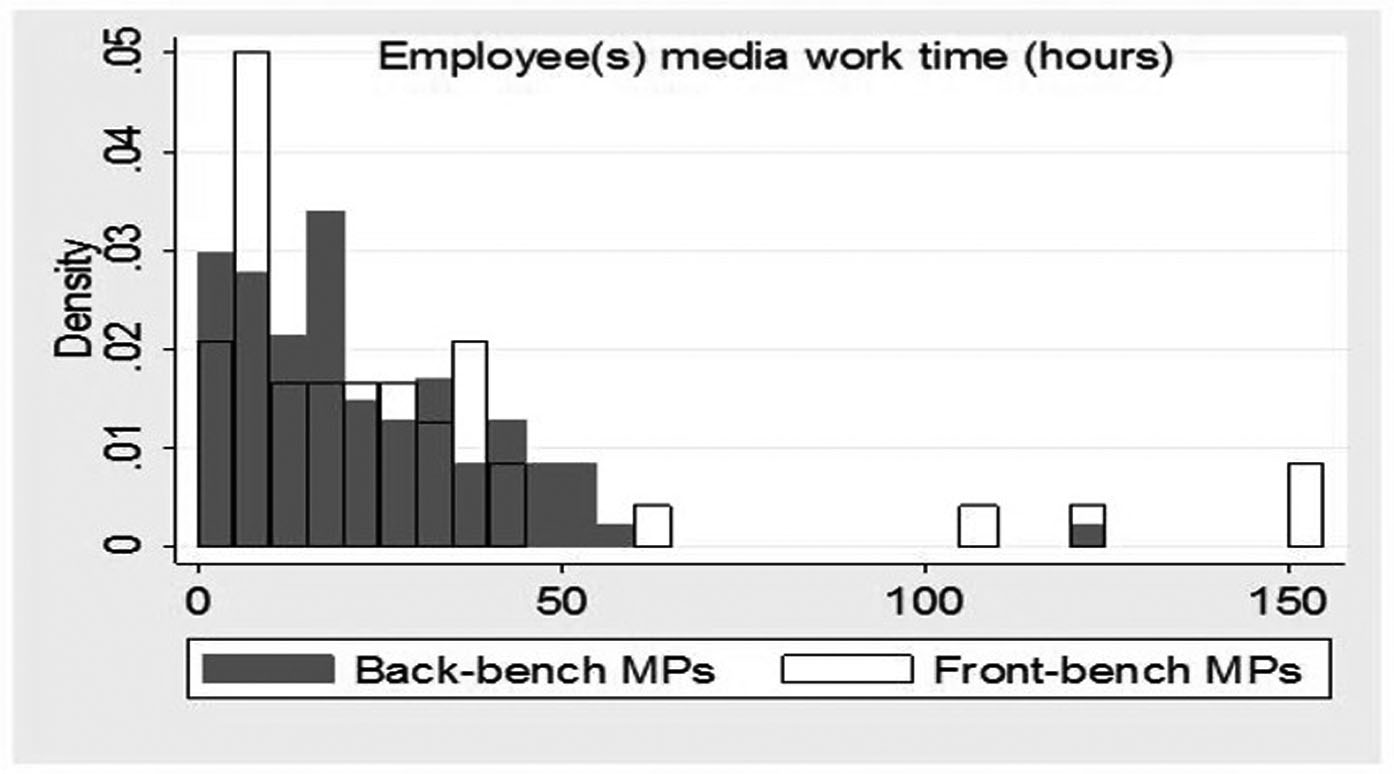The image features a detailed graph titled "Employees' Media Work Time (Hours)." The y-axis represents density, scaling from 0 to 0.05, while the x-axis features intervals at 0, 50, 100, and 150 units, though the exact nature of these units is unspecified. The graph differentiates between two categories of MPs (Members of Parliament): backbench MPs, depicted with black bars, and frontbench MPs, illustrated with white bars. The graph suggests that frontbench MPs demonstrate higher density values near 0.01. This observation is contrasted with backbench MPs, who are represented less densely. Overall, the background of the graph is white, and it is framed in a grayish-beige border.